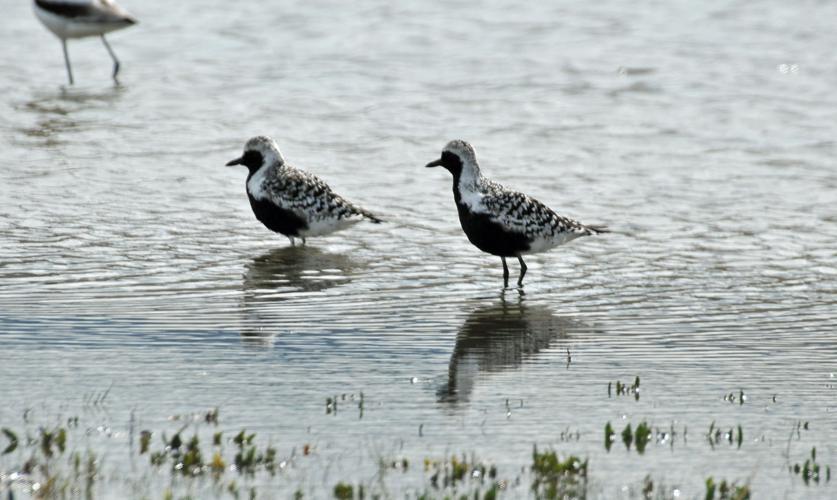This is a detailed photograph capturing a serene scene in a shallow salt marsh. Dominating the center of the frame are two birds standing side-by-side in the water, both facing left. These birds exhibit distinctive plumage: white heads with black mottling, black beaks, black faces, and black bellies. Their white backs also feature black speckles. The water stretches across the entire frame, showing subtle ripples and reflecting the birds' shapes. In the foreground, small patches of grass poke through the water, adding depth to the scene. Additionally, in the top left corner, there is a partially visible bird, likely a different species, with only its body and legs discernible as its head is cut off and it appears blurred.